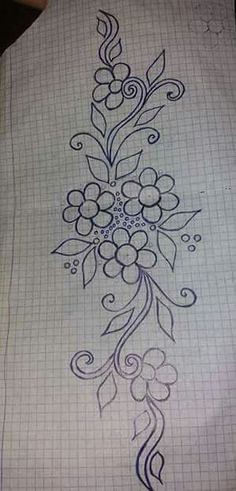This detailed close-up photograph captures a drawing on graph paper, characterized by its grid of small squares created by black horizontal and vertical lines. On the left side, a dark blue vertical line intersects some of these squares. The artwork itself is a carefully rendered floral pattern, suggesting it could be a tattoo outline. At the center of the composition are three primary flowers, each with six egg-shaped petals and a circular core, arranged in a triangular formation. These flowers are connected by swirling, vine-like branches, adorned with diamond-shaped leaves and teardrop-shaped leaves.

The intricate design extends horizontally, with both the top and bottom of the image featuring additional curly branches, floating diamonds, and smaller flowers. Notably, a top-right section shows hexagonal shapes, possibly an area where the artist practiced their technique, and a partially drawn flower with four petals. The entire drawing is executed with a blue pen, resulting in various levels of line thickness and intensity, suggesting different stages of fading. Dotted areas in the middle, along with carefully placed circles and partially colored shapes, add to the complex texture of the design, making it appear both meticulously detailed and organically flowing.